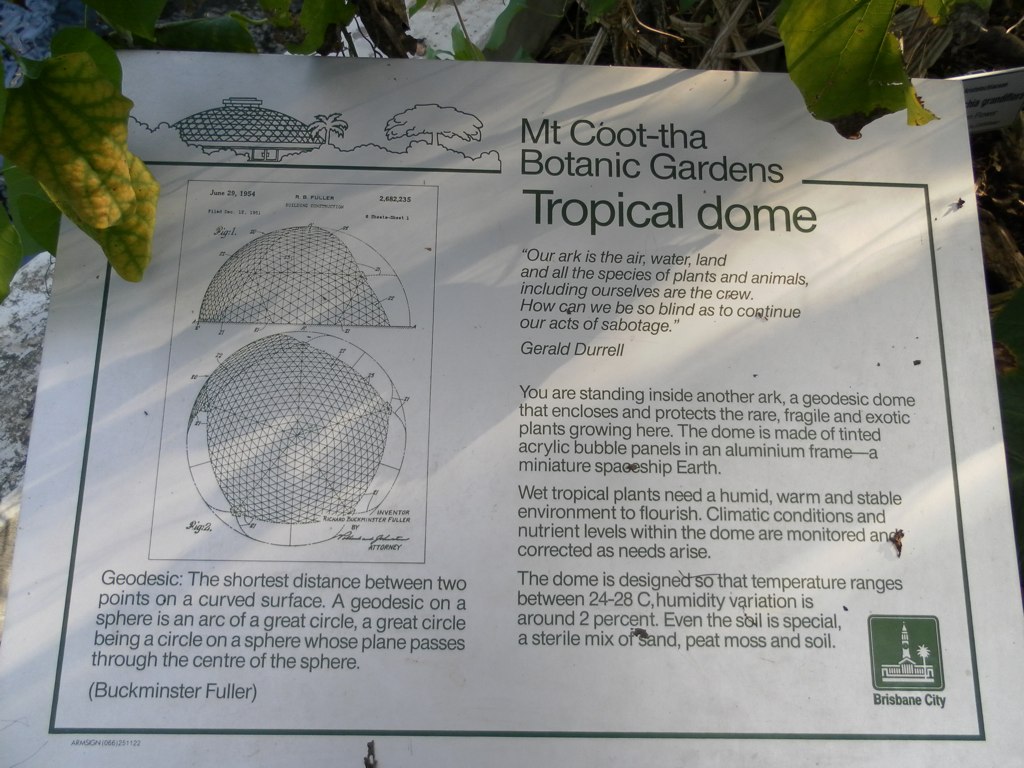The image depicts a white plaque with green text, set outdoors near the ground, surrounded by branches and leaves. The plaque, viewed from a top-down angle, provides detailed information about the Tropical Dome at the Mount Coot-tha Botanic Gardens in Brisbane City. The top of the plaque is adorned with an illustration of the dome, while the left side features a three-dimensional diagram of the dome, along with a definition and explanation of the term "geodesic" by Buckminster Fuller. The right side of the plaque includes a quote by Gerald Durrell: "Our ark is the air, water, land, and all the species of plants and animals, including ourselves, are the crew. How can we be so blind as to continue our acts of sabotage?" Below the quote, there are detailed descriptions of the dome, stating that it is a geodesic dome made of tinted acrylic bubble panels in an aluminum frame, designed to create a humid, warm, and stable environment for rare, fragile, and exotic wet tropical plants. The text highlights the controlled climate conditions within the dome, maintaining temperatures between 24-28°C and humidity variation around 2%. The soil inside the dome is a special, sterile mix of sand, peat moss, and soil. At the bottom right of the plaque, there's a stamp bearing the text "Brisbane City" and an accompanying icon.